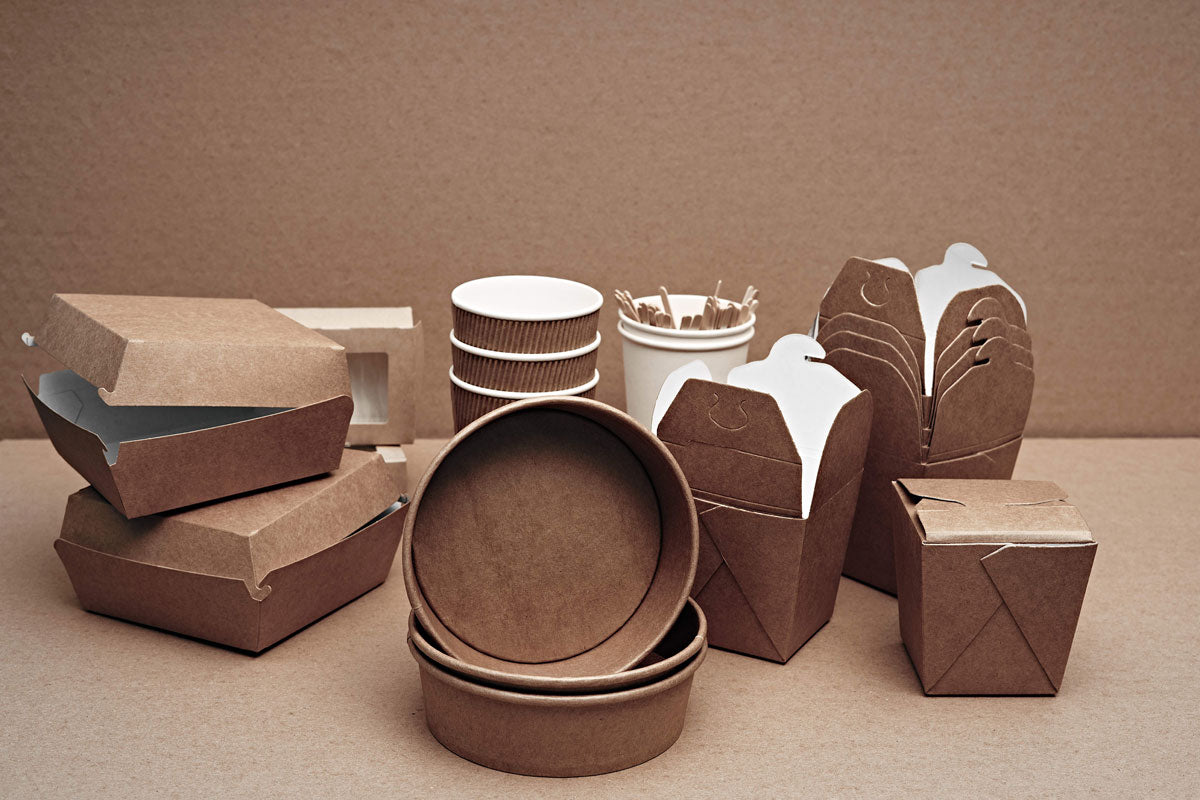The photograph features a professionally arranged display of various restaurant takeout containers, all set against a brown background that resembles a wooden table. The containers are predominantly made of cardboard or paper. On the left side, there are brown cardboard boxes ideal for sandwiches or hamburgers, showcasing white interiors. Moving right, there's a stack of corrugated brown cups with white insides, alongside white coffee cups adorned with brown stars, each containing wooden stirring sticks. At the forefront are bowl-shaped containers, all with a brown exterior and white interior. To the far right, traditional Chinese takeout boxes with folding tops are also clearly visible, in matching brown and white colors. The well-lit setting, devoid of any text, suggests that this image is likely intended for a website targeting food distributors or restaurants looking to purchase disposable takeout containers in bulk.